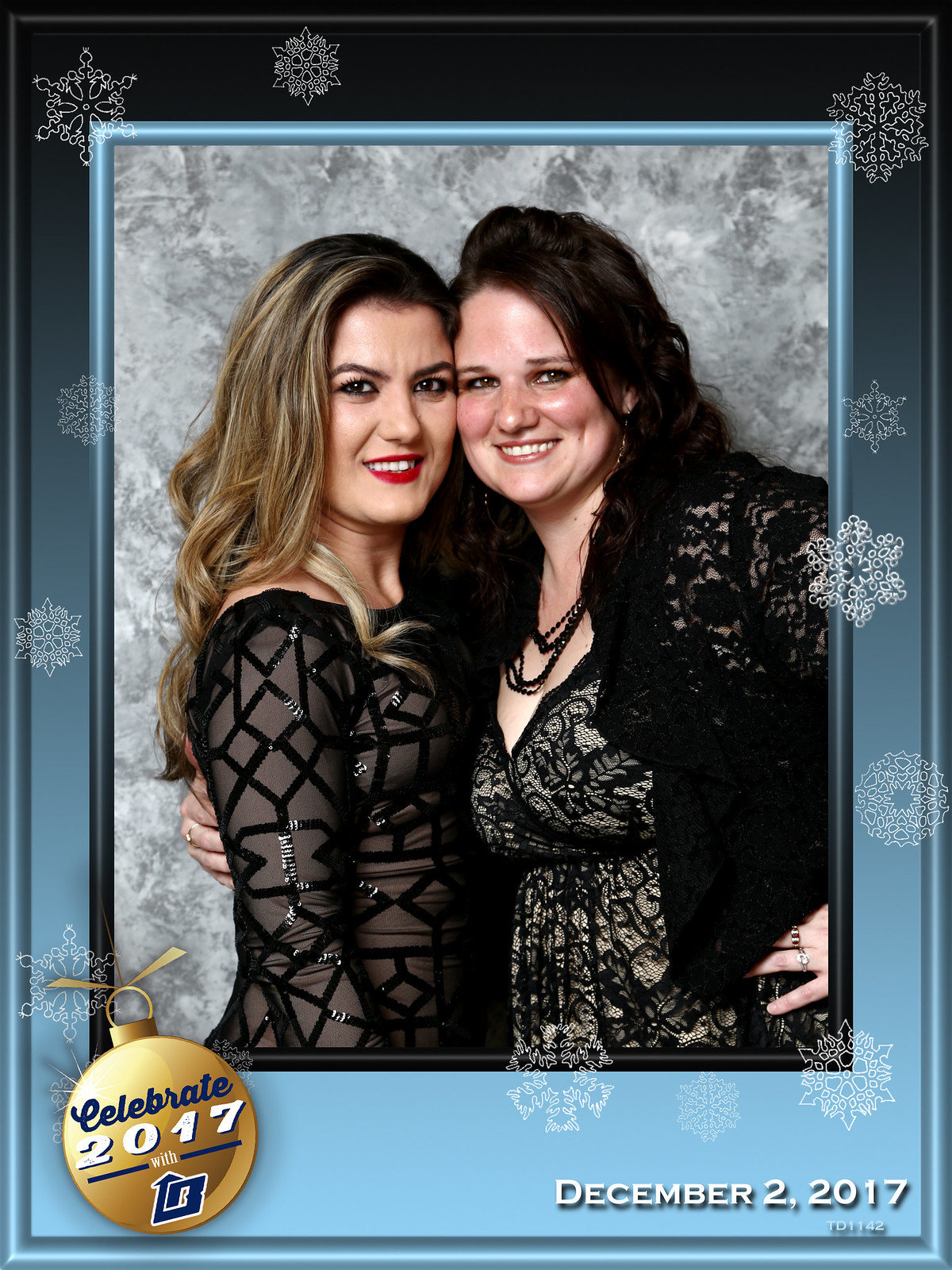This portrait photograph, taken on December 2, 2017, is of two Caucasian women standing closely together against a gray, snowy-looking backdrop. They are cheek to cheek, smiling warmly at the camera. The woman on the left has long, dark brown hair with blonde highlights in loose curls cascading past her shoulders. She wears bright red lipstick, dark eye makeup, and has dark brows over her intense gaze. Her outfit is a sheer black top adorned with black stripes and patterns. The woman to her right, slightly paler, has long, dark brown hair, though the length isn't entirely visible. She is dressed in a black lace dress paired with a black beaded necklace and a matching lace shawl. Her broader smile reveals a happy demeanor, and her arm is affectionately wrapped around the first woman, with her other hand resting on her hip. The border of the photograph features a gradient from light blue at the bottom to midnight blue at the top, embellished with white snowflakes around the edges. In the lower left corner, there is a gold Christmas ornament with the inscription "Celebrate 2017" alongside a logo. The date "December 2, 2017" is printed in white in the bottom right corner.